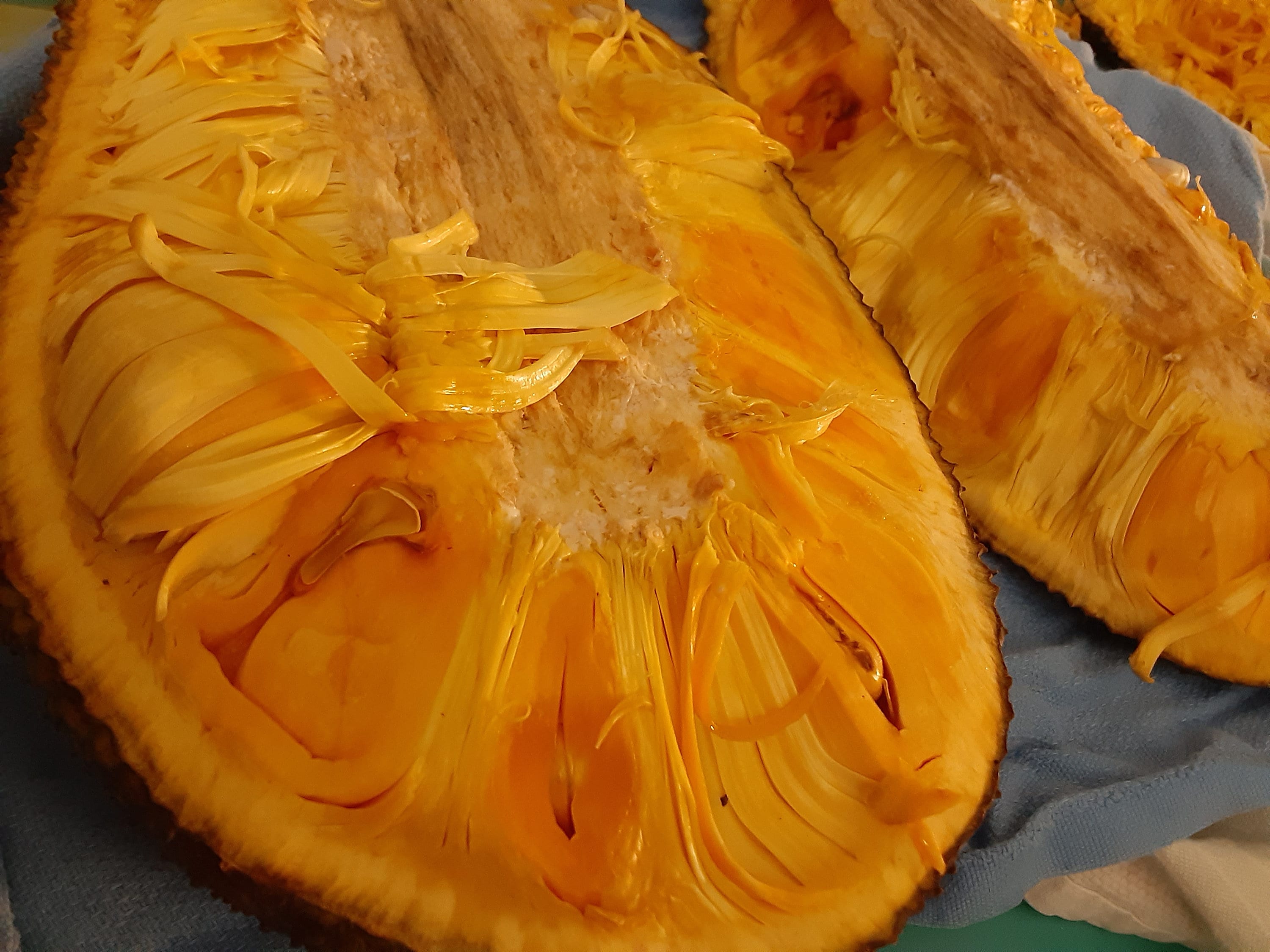The image depicts a close-up of what seems to be a dried or cut-open yellow-orange melon or squash, potentially a spaghetti squash. The fruit, with its vibrant yellow, fibrous, and stringy interior, is positioned atop various layers, starting with a blue fabric, followed by a white cloth and then a teal cutting board. Three pieces, halved and laid side by side, reveal their interiors with some seeds visible amidst the fibrous pulp and an orangey core. The rough, craggy exterior contrasts with the rich, textured inside. In the background, there are additional slices showing parts of the seeds and fruit pods.